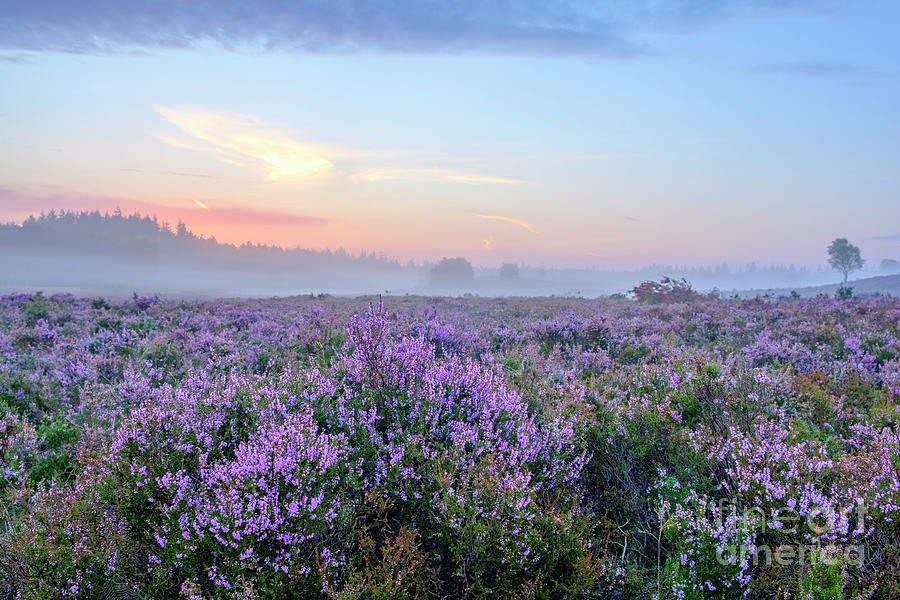A captivating photograph captures an expansive field of purple lavender stretching as far as the eye can see. Amidst the lavenders, occasional patches of orange and green grasses add diversity to the landscape. Dominating the scene is a particularly tall lavender flower near the center of the image. The sky above is adorned with swirly white clouds and drenched in the warm hues of a setting sun, blending shades of blue, orange, pink, and red. To the left, a dim forest is hazily visible through the fog, and scattered trees punctuate the meadow. In the far background, the silhouette of mountains adds depth to this picturesque setting. The photograph bears a watermark on the bottom right corner, reading "Fine Arts America," with 'Fine' in a delicate thin font and 'Arts America' in a bold font, underscoring its professional quality.